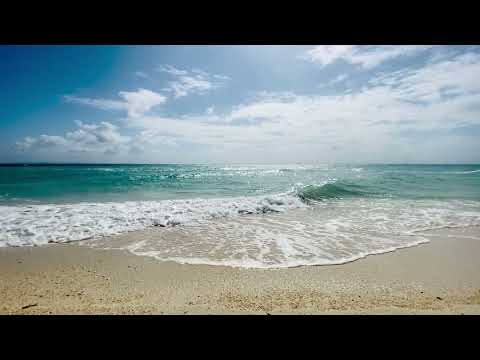This photograph captures a serene daytime beach scene viewed from the shoreline. The foreground is dominated by smooth, wet sand of a light beige to golden color, still glistening from the gentle waves. These waves crash against the shore, creating a thin sheet of white, frothy water filled with oxygen bubbles. The ocean water, a striking greenish teal, extends towards the horizon where cross-wave action is noticeable, with some waves running perpendicular to the beach. Above the teal ocean, the sky is a brilliant blue, adorned with scattered white clouds. The image itself appears to be a screengrab, evidenced by the horizontal black borders on the top and bottom of the frame, likely indicating it's viewed on a digital screen.